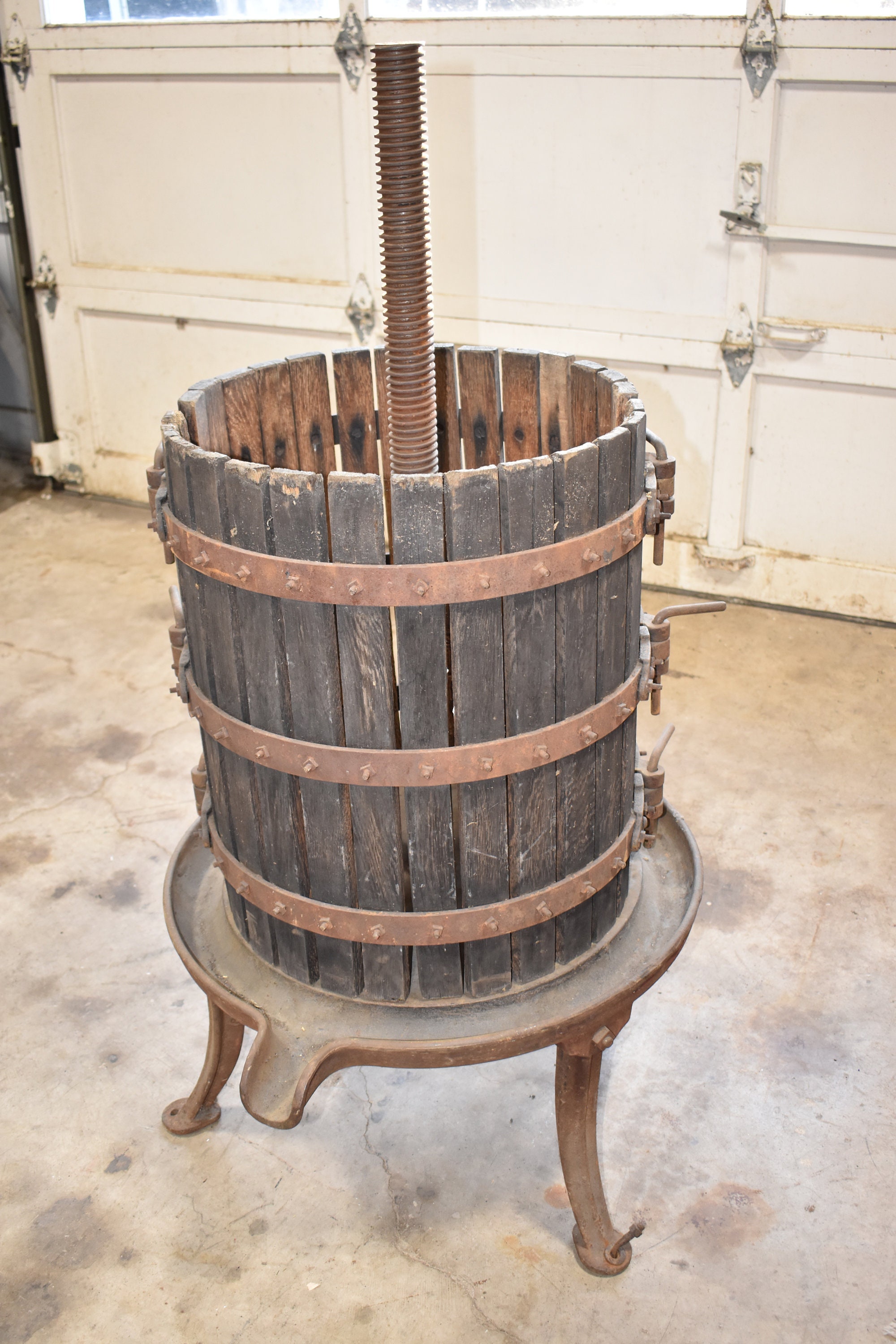In this detailed indoor daylight photograph of a garage, the main subject is an antique wooden barrel mounted on a sturdy, metal platform. The concrete floor below is light tan with brownish spots, enhancing the rustic aesthetic of the scene. The background features part of a white garage door with metal handles. The barrel is composed of vertically aligned dark brown wooden staves, tightly bound by three rusty copper-colored metal hoops. A prominent metal screw mechanism extends from the top of the photograph down into the center of the barrel, indicating that this is likely an old-fashioned press, possibly for apples or other fruits. The barrel sits on a bronze-colored metal base with multiple legs and a short spout on the front left, designed to drain the extracted juice into a waiting receptacle. The scene captures the timeless essence of traditional craftsmanship within the utilitarian setting of the garage.